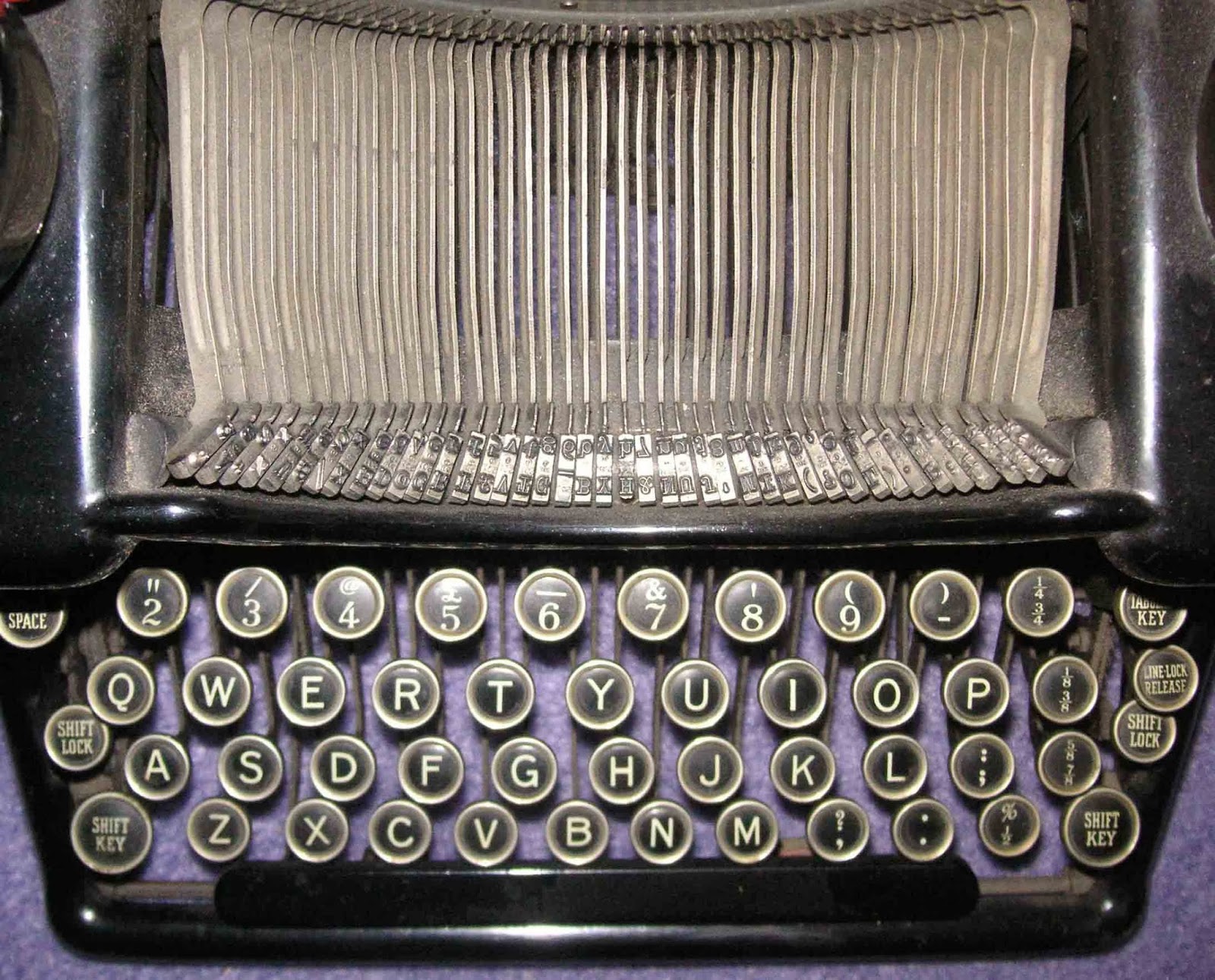This full-color, square photograph, taken indoors under artificial lighting, captures an old-fashioned, manual typewriter displayed on a purple countertop. The typewriter, possibly from the late 19th or early 20th century, features a traditional QWERTY keyboard with round, white-lettered keys bordered in black. The detailed view exposes the intricate inner mechanics of the machine while omitting the platen. The top row includes the letters Q through P, followed by A through L in the middle row, and Z through M on the bottom row. Notably, the typewriter's numerical keys span from 2 to 9, lacking a number 1. Both shift keys, the space key, a distinctive round button for uppercase, and additional function keys such as shift lock and line lock, are present. The black body of the machine indicates it was likely used as an office typewriter and would be familiar to those who have experience with manual typewriters.